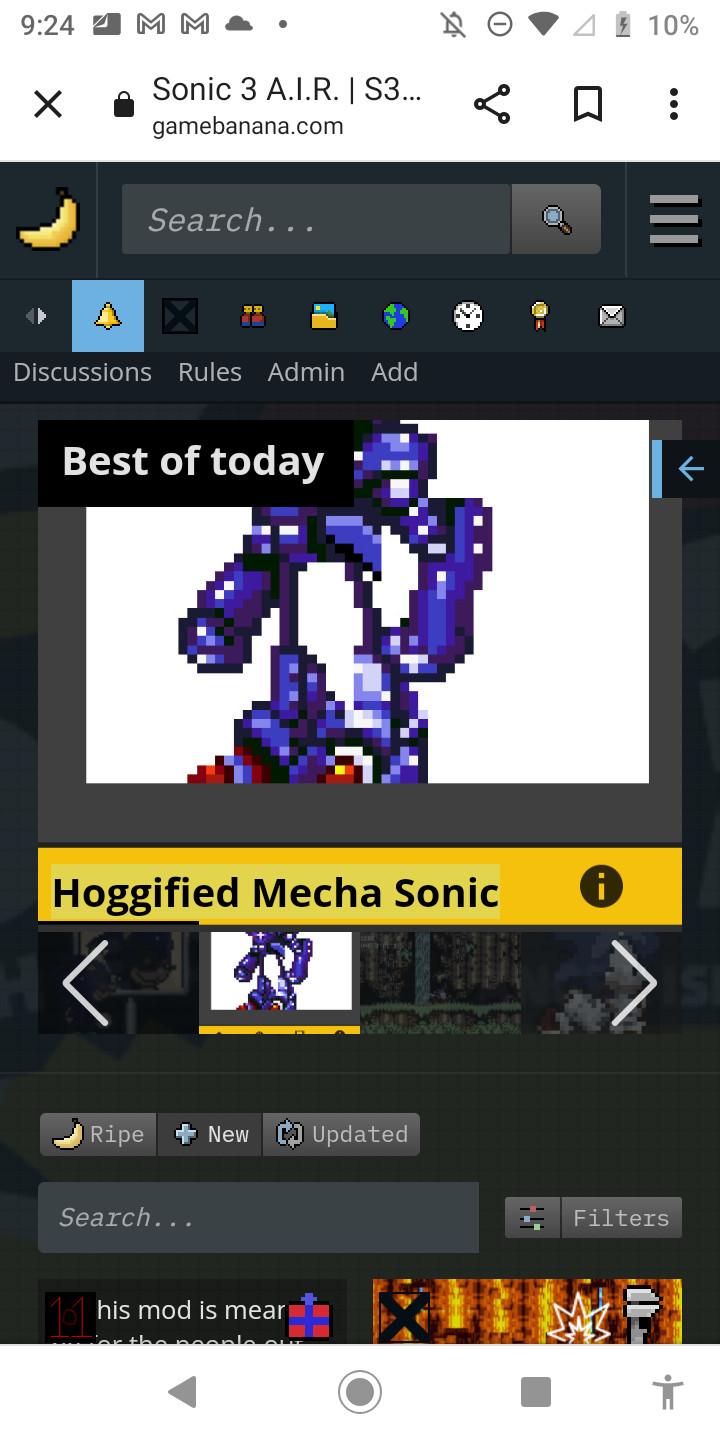The image is a screenshot of a game-related app or website displayed on a smartphone. The interface has a pixelated aesthetic, likely reminiscent of a 16-bit style. In the upper left-hand corner, there is an icon resembling either a crescent moon or a banana, next to which is a gray search bar with the italicized word "search..." followed by three dots. To the right of the search bar is a magnifying glass icon, and further right, aligned to the edge of the screen, is a hamburger menu represented by three horizontal lines.

At the top of the screen, the time is shown as 9:24, accompanied by various status icons: two Google icons, a cloud icon, a Do Not Disturb bell with a line through it, a circle with a minus (possibly a notification indicator), a Wi-Fi signal icon, a phone signal icon, and a battery icon showing 10% charge. 

Below these icons is a prominent header with an 'X' on the left. Centered on the screen is the text "Sonic 3 A.I.R." followed by a separator line, the text "S3..." with three dots, and "GameBanana.com". Directly below the search bar are various icons, including a highlighted bell icon.

The main content area features a section labeled "Best of Today", with a highlighted item "Hogafied Mecha Sonic" under an image. This section includes a carousel display, allowing users to scroll through different highlighted items. Below the carousel are several buttons labeled "Bright," "New," and "Updated," along with additional search and filter options to refine content selection.